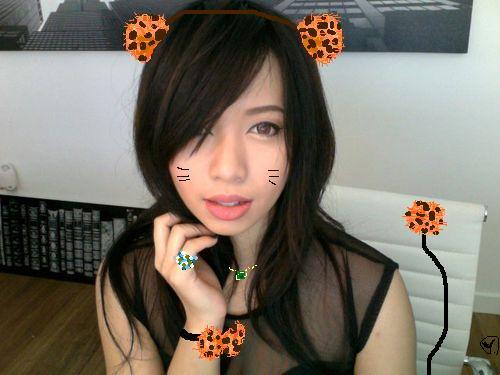The photograph features a close-up shot of a young Asian woman, approximately 19 years old, with fair skin and long black hair with bangs partially covering one eye. She has brown eyes, adorned with eyeliner, and is wearing an orange leopard-print headband with cat ears and a matching bracelet. Whiskers are artistically drawn on her cheeks, contributing to her cat-like appearance, enhanced by the illusion of a tail in the same leopard-print design. She is dressed in a black, sheer mesh top, partially see-through, and is seated on a white chair. Her right arm is raised to rest underneath her chin, and her mouth is slightly open. The background reveals a white wall with some design elements, including what appears to be the bottom half of a picture of buildings and a monochromatic image of books. A small table is also visible, reinforcing the indoor setting of the room.